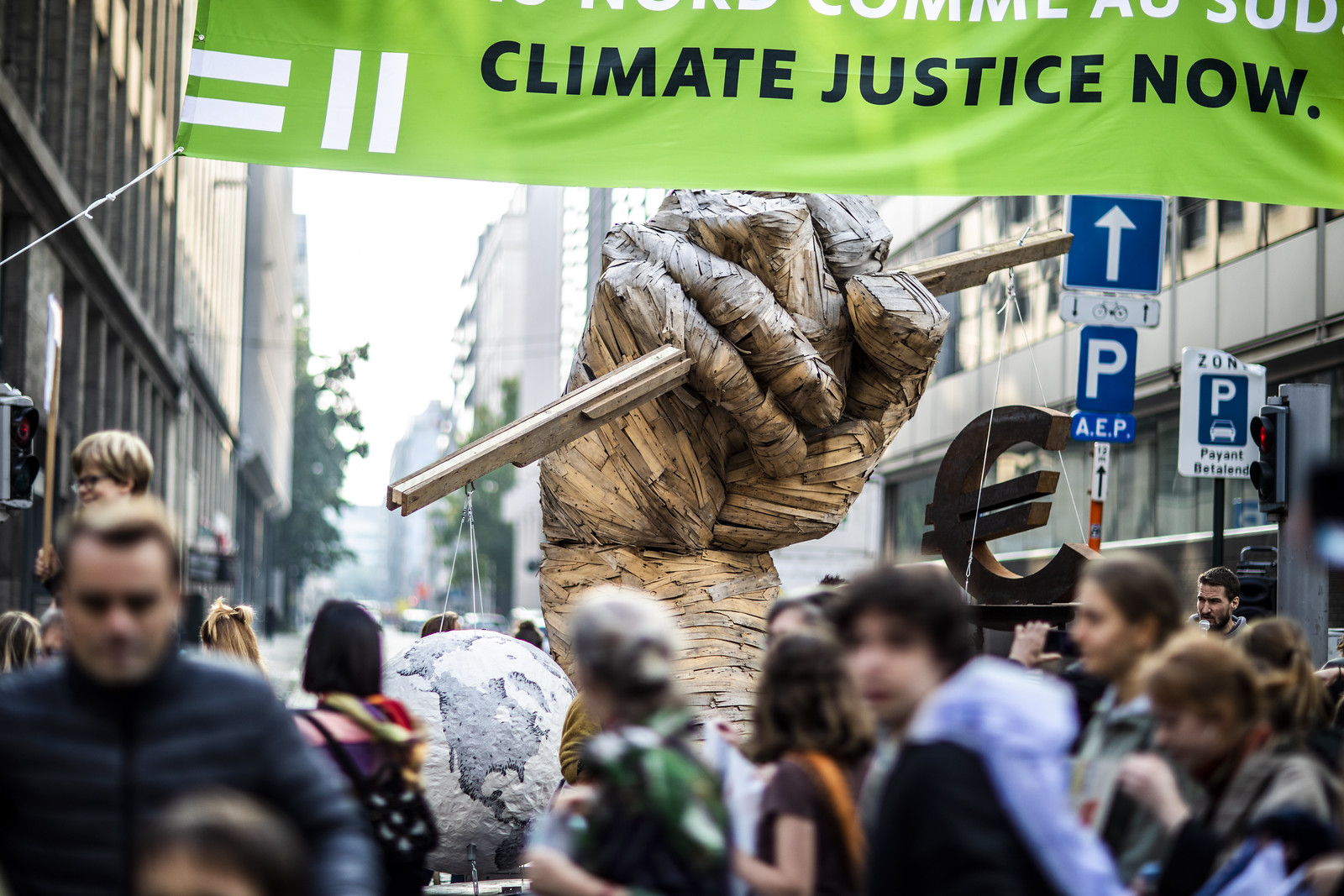The image depicts a detailed and elaborate art installation situated in a bustling city square. A towering statue of a fist, meticulously crafted from scraps of wood, holds an old-fashioned balance scale. This scale features a globe on the left side and a Euro symbol on the right, with the globe weighing down and tipping the scale in its favor, symbolizing the greater importance of the Earth over monetary concerns. Above the statue hangs a prominent light green banner with white stripes, inscribed with the bold message "Climate Justice Now," although additional text at the top of the banner is obscured. The scene appears to be a peaceful demonstration rather than an active protest, as various individuals, blurry and diverse in age and gender, are either gathered around the installation or walking by. The surrounding urban environment consists of tall buildings on either side, and blue parking signs are visible, indicating a downtown area that could be the European equivalent of Wall Street. The sky above the buildings appears white, leaving its actual color undetermined.